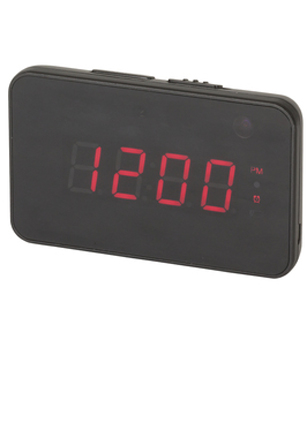A sleek and modern alarm clock is showcased in this minimalistic image. The design features a thin, black, rounded rectangle that is reminiscent of a smartphone in size. The alarm clock is displayed in a horizontal landscape orientation, emphasizing its streamlined profile. Its digital display prominently shows the time as "12:00" in bold red numbers, with a subtle "PM" indicator in small letters to the right, confirming the time of day. Additional icons are faintly visible on the right side of the display, adding to its functionality. At the top of the alarm clock, two buttons are discernible, with one likely being a snooze button. This entire device is set against a pristine, pure white background, which lacks any additional detail, suggesting that this may be a product shot or a CGI rendering designed to highlight the clock's modern and minimalistic design.